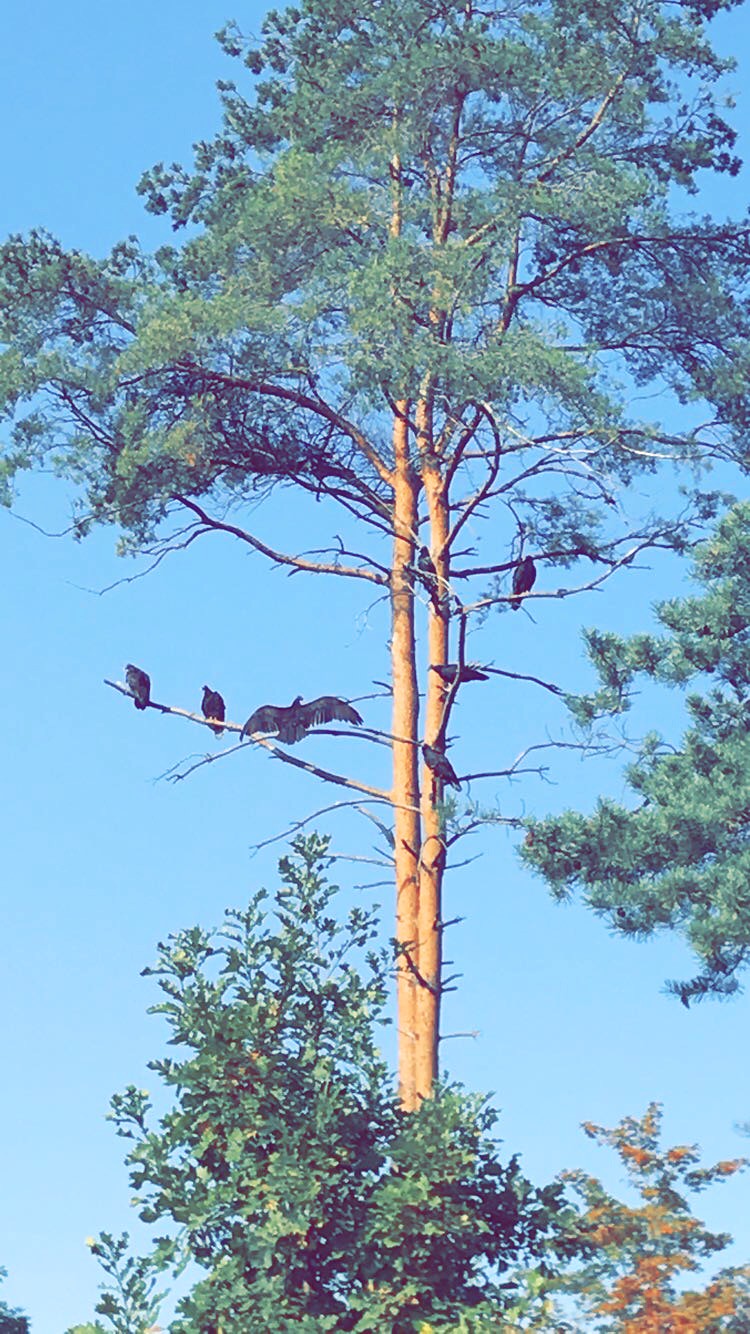In this image, a tall, narrow tree stands prominently in the frame, seemingly fused at its base with a neighboring tree by a dense bush, obscuring the bottom portion. The tree, with its exposed bark stretching high up until it reaches a sparse canopy of green leaves, hosts seven birds perched throughout its branches. The birds, likely black eagles or crows, dot the tree: one bird is seen with its wings outstretched as if sunbathing, while the others sit separately or in small clusters on various branches. The sky is bright blue, offering a striking backdrop, and other green bushes and trees can be seen nearby, enhancing the lush setting.